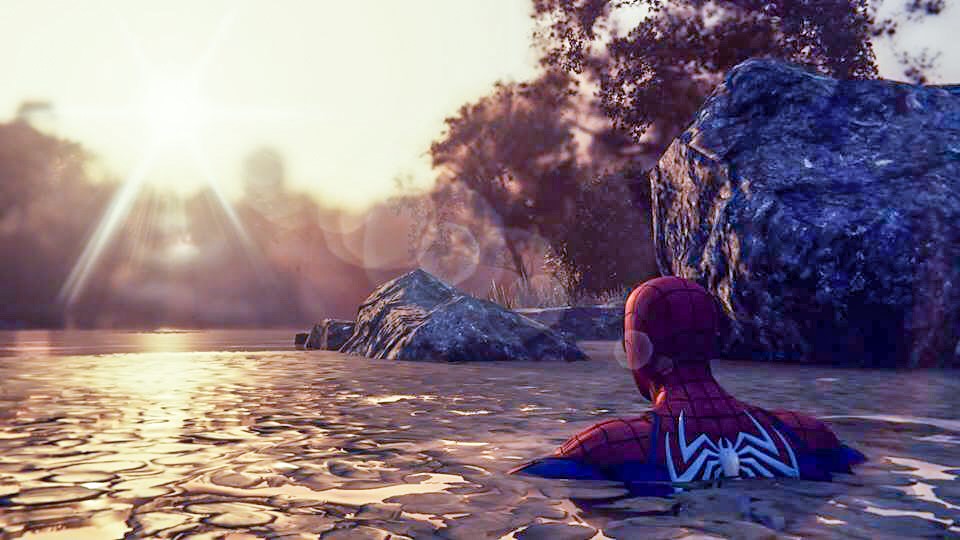A digitally-created image depicts Spider-Man relaxing in a spring, with only part of his iconic suit visible. The white spider emblem is prominently displayed on his back, while sections of his blue costume and the red mask on his head are discernible. The red mask features a pattern of squares, adding intricate detail to his appearance. A lens flare effect enhances the middle of the image, contributing to the scene's vividness. The water Spider-Man is in appears slightly murky due to algae-like substances floating on the surface. To his left, a gray and white rock outcropping is visible, providing a natural backdrop. A leafy tree stands near the spring, with rays of sunlight piercing through the foliage and reflecting off the water, creating a serene and picturesque setting.